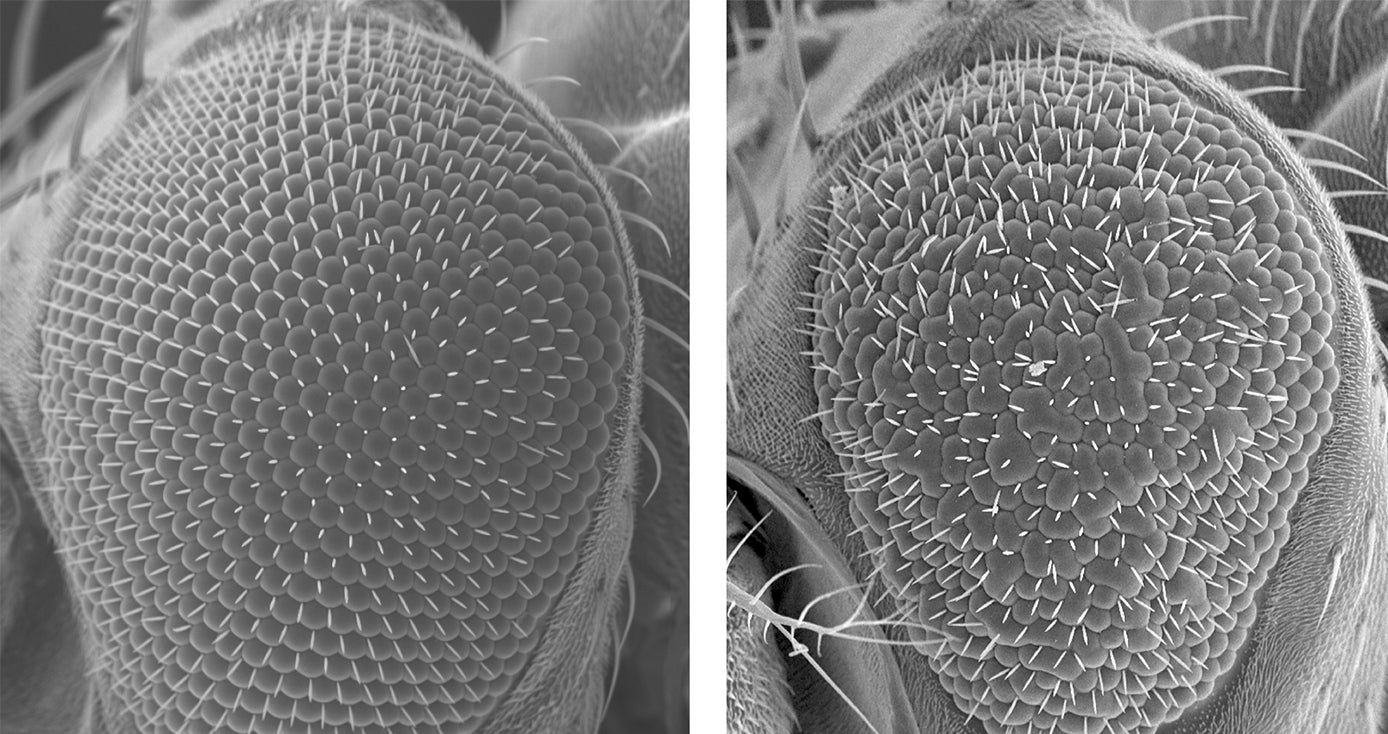This grayscale image features two side-by-side abstract images, likely microscopic views, portraying intricate organic structures. Both images depict plant-like or biological forms, possibly resembling a thistle, cacti, or a fly’s eye, with a dense configuration of cells and spiky hairs. The left image displays a more structured arrangement with thistle-like protrusions confined within the object. In contrast, the right image shows a chaotic scene with more pronounced, protruding spikes and wrinkled, less organized cells. The entire composition is rendered in shades of gray, evoking an impression of a deep, magnified view perhaps using advanced imaging techniques to reveal the detailed surface textures and cellular patterns.